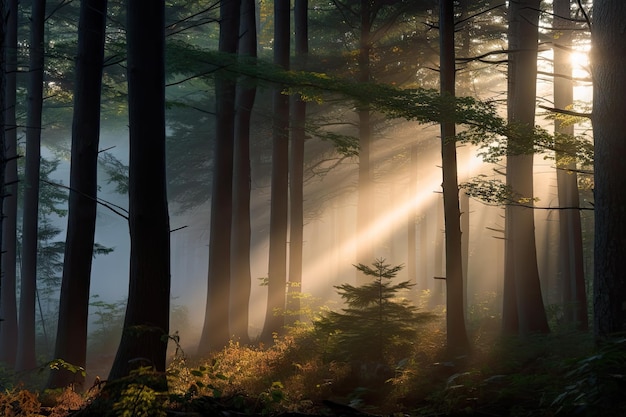This photograph captures a deep and dense forest scene characterized by tall, slender tree trunks rising high with their branches primarily towards the top, forming a thick evergreen canopy intermixed with substantial foliage. The ground is dotted with a variety of growth, including waist-high saplings, smaller shrubs, and patches of orangish-brown plants, adding a level of detail to the forest floor. The sun, situated in the upper right corner, casts striking rays through the trees, which start vividly and become more diffused as they descend towards the bottom left of the image. This sunlight filters through the foliage, creating a beautiful interplay of light and shadow and illuminating the otherwise dark and somewhat misty forest, contributing to the scene's ethereal and serene atmosphere. Bold sunbeams in the image cut through the fog and darkness, providing a stark contrast that brings warmth and a touch of brightness to the muted colors of the forest.